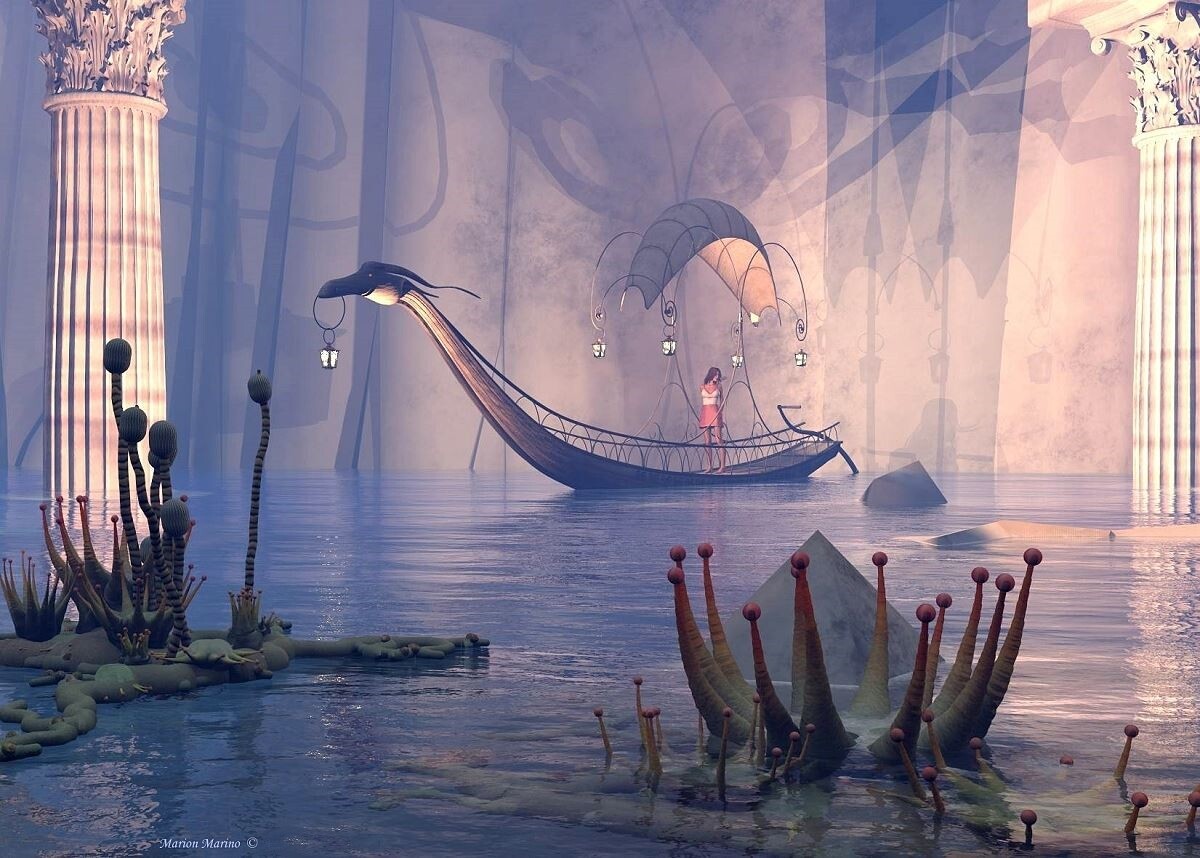The image depicts an intricate and atmospheric scene of a gondola-like boat floating on a body of water within a subterranean or castle-like concrete structure illuminated by pillars. The gondola, adorned with a front resembling a water dragon or bird's head, grips a lit lantern in its mouth. The vessel is covered by a tarp arching over the top, presumably shielding the solitary female figure standing in the middle. The boat is bordered by a net railing, and although the steering pole is visible, there's no one at the helm. The water around the gondola is populated with green, floaty vegetation and odd-shaped plants, alongside jagged rocks or platform bases for the pillars. Shadows cast by the structures and light create a mysterious and enchanting ambiance.